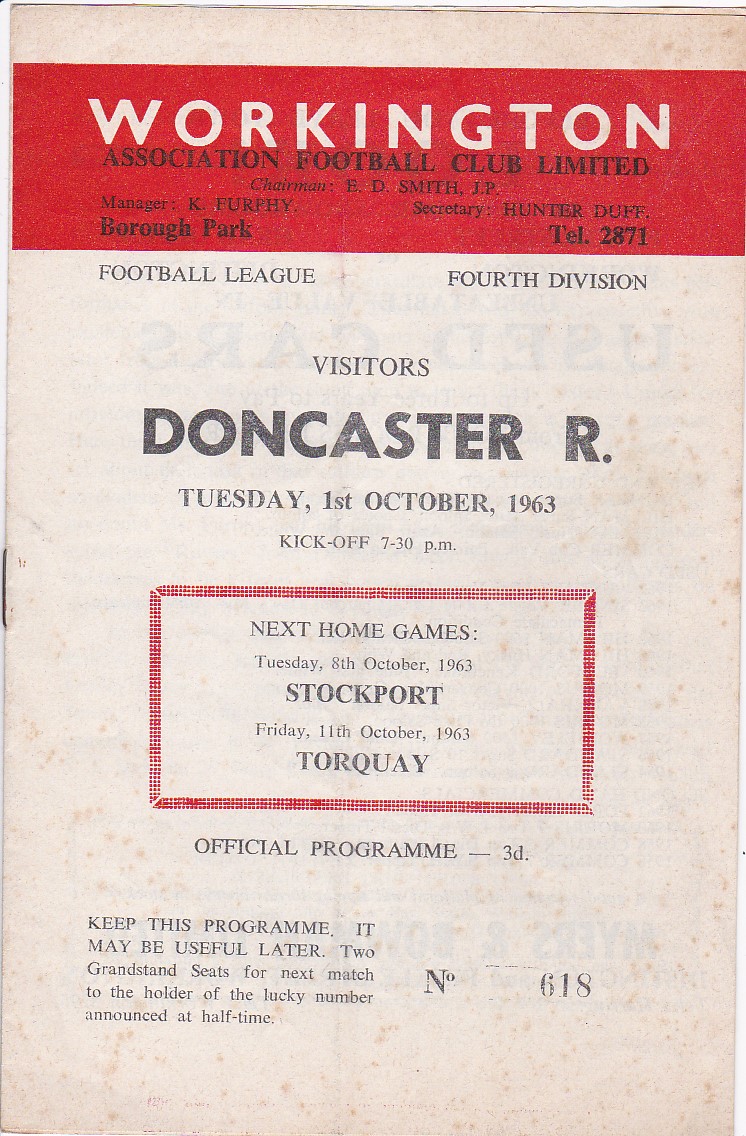The image depicts the front cover of an aged, vintage program for an upcoming football match from 1963. The program is for Workington Association Football Club Limited, prominently featuring tan, red, white, black, and grey colors. At the top is a red horizontal banner with white text stating "WORKINGTON," followed by black text declaring "Association Football Club Limited." It lists key personnel: Chairman B.D. Smith, Manager K. Turfey, and Secretary Hunter Duff, along with contact information.

The central section contains bold black text: "VISITORS: DONCASTER R.," underlined by the date and time "TUESDAY, 1st OCTOBER 1963, Kickoff 7.30 pm." Below this is a red-bordered rectangle highlighting upcoming games, including Stockport on Tuesday, 8th October, and Torquay on Friday, 11th October.

The bottom part of the cover features a note: "Official Program 3D," and advises to keep the program for potential usefulness later. A unique identifier "No. 618" appears on the right. The cover shows signs of age, like dirt marks and an old staple on the left side, exemplifying its vintage print publication style. The program fully occupies the image, emphasizing its historical significance for a sports event held in Bureau Park, part of the Football League's Fourth Division.